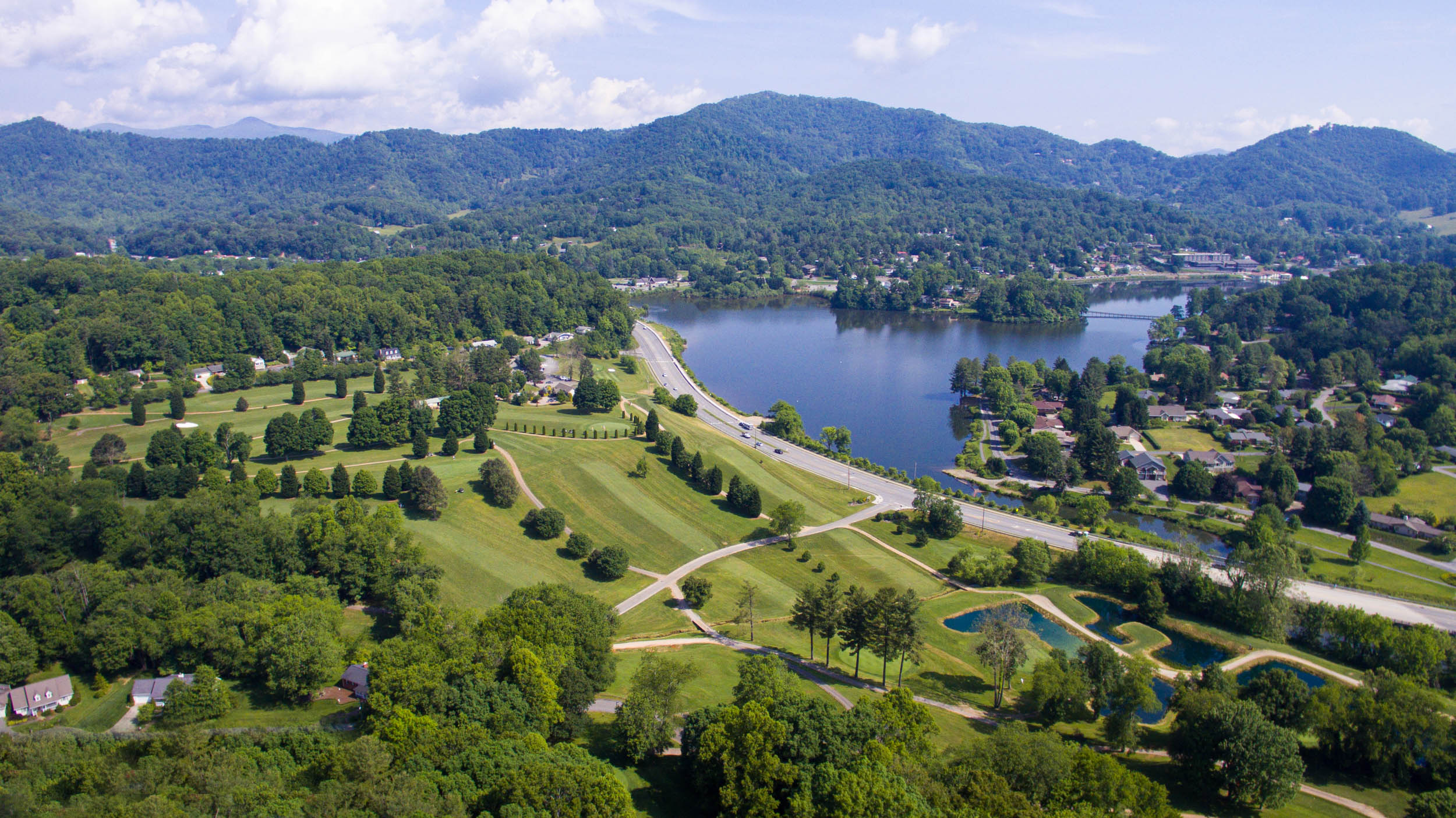This aerial photograph captures a picturesque landscape centered around a meticulously maintained golf course situated by a serene lake. The image is framed by lush greenery and features a sprawling golf course on the left side, complete with neatly cut paths for golf carts and sparse clusters of trees. Towards the bottom of the picture, a dense thicket of trees resembles a forest, surrounding several houses, particularly concentrated in the bottom left corner. A long street runs diagonally from the top left center toward the bottom right corner, intersecting with additional roads that diverge to connect various houses both above and below the main thoroughfare. In the distance, a bridge spans the lake, linking two forested sections. Beyond the bridge, more buildings dot the landscape, extending towards gently rolling, tree-covered hills. An interstate separates the golf course from a series of smaller interconnected lakes to the right, where the golf course continues and even features a small island. This idyllic scene, with its expansive, well-manicured lawns and scattered homes, conveys an air of affluence and tranquility.